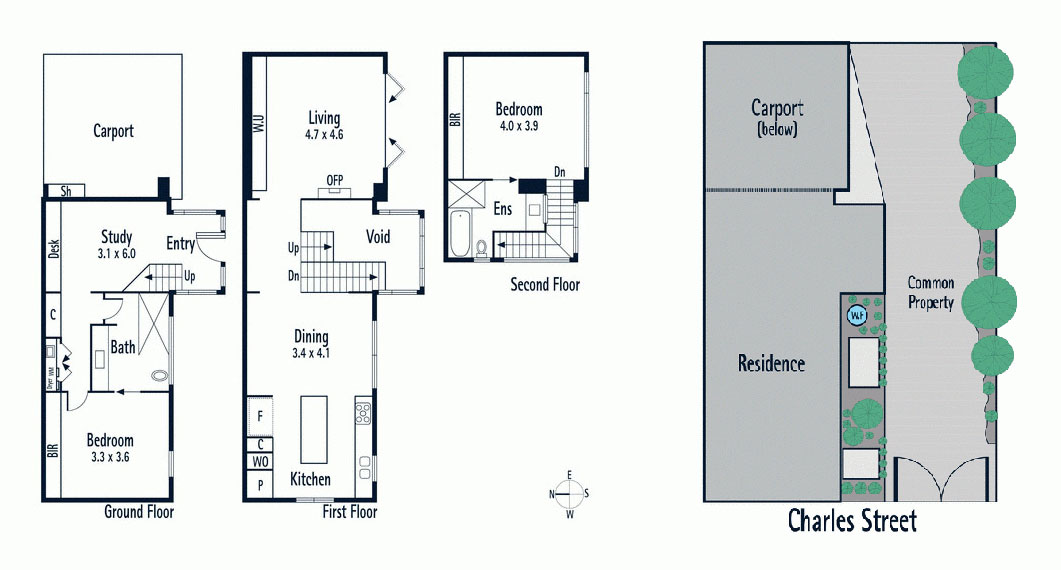This image features a detailed architectural plan, divided into two sections on either side. 

On the right-hand side, there's a general blueprint of a property located on Charles Street. This outlines a carport positioned at the top, beneath which lies the main residence. Adjacent to the right of the residence is an area marked for greenery and several outdoor structures, although the specific purposes of these buildings are not indicated. Further right, the blueprint depicts a common property area accessible through a double gate. This common property is bordered by a line of trees on the right-hand side of the property layout.

The left-hand side of the image provides a more detailed blueprint of the residence. It includes floor plans for the ground floor, first floor, and second floor. On the ground floor, starting at the top of the blueprint, there's a carport. Next to the carport is a study measuring 3.1 by 6.0 units (units not specified). The study contains a designated area for a desk and is accessible via an entrance from the outside. Within the study, there's a staircase leading up to the higher floors. Continuing from the study, the blueprint shows a bathroom equipped with a bath and a toilet. Past the bathroom, you arrive at a bedroom measuring 3.3 by 3.6 units, which appears to have a window or possibly a door leading outside.

Ascending to the first floor, the area above the carport serves as the living room, which connects through a hallway to a combined dining room and kitchen space. The kitchen features a central table or large counter. Stairs provide access to both the ground floor and the second floor.

On the second floor, situated above the carport and living room, is another bedroom, complete with an en suite bathroom. The en suite includes a bath, toilet, and sink.

Overall, the image combines both a general property layout and a specific, detailed architectural plan of a residence, offering a comprehensive view of the entire property on Charles Street.